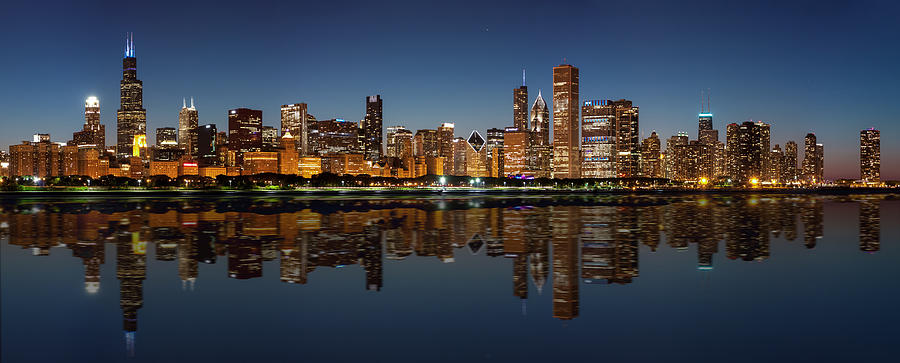The photograph captures a panoramic view of a vibrant city skyline at dusk, transitioning into night. Dominated by a deep blue sky that fades to cyan, the towering skyscrapers and smaller buildings are illuminated, their lights reflecting brilliantly off the dark blue water below. This creates a serene yet striking mirrored image of the skyline. On the right side, the last traces of the sunset add red splotches to the darkening sky. Notably, one skyscraper on the left side is adorned with purple and blue spirals at its top, adding a unique touch to the cityscape. The scene likely depicts the Chicago metropolitan area, featuring numerous illuminated skyscrapers, some topped with needles and one prominent diamond-shaped building in the center.